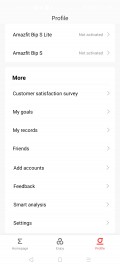A screenshot of a mobile device's settings window titled "Profile" at the top. The majority of the text is blurry and unreadable. However, beneath the title, readable bolded text includes the word "More," followed by "Customer Satisfaction," "Delivery," "Michaels," "Friends," "Ad Accounts," and "Settings." There appear to be additional options that are illegible due to the blurriness of the image. At the bottom of the screen, there are three tabs; the one on the far right is red, while the other two are black, matching the black text of the profile settings window.